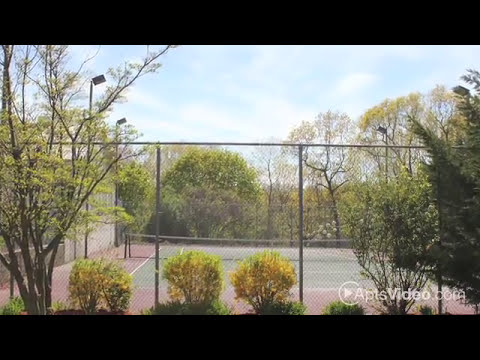The image captures an outdoor scene on a clear, early spring day, defined by a blue sky dotted with white clouds. The top and bottom are bordered by black rectangular stripes, and the lower left corner features the text "aptsvideo.com" alongside a play button icon. Prominently featured is a tennis court, enclosed by a tall, chain-link fence, approximately 20 feet in height. The court surface is green, framed by a reddish-brown perimeter, with a net stretching across its center. Surrounding the court, a dense array of deciduous and evergreen trees, some budding with new leaves and small yellow flowers, evokes a vibrant, natural setting. Tall lights loom over the scene, presumably for night play. Bushes and other flora add to the rich, earthy palette dominated by greens, maroon, and touches of yellow and silver.